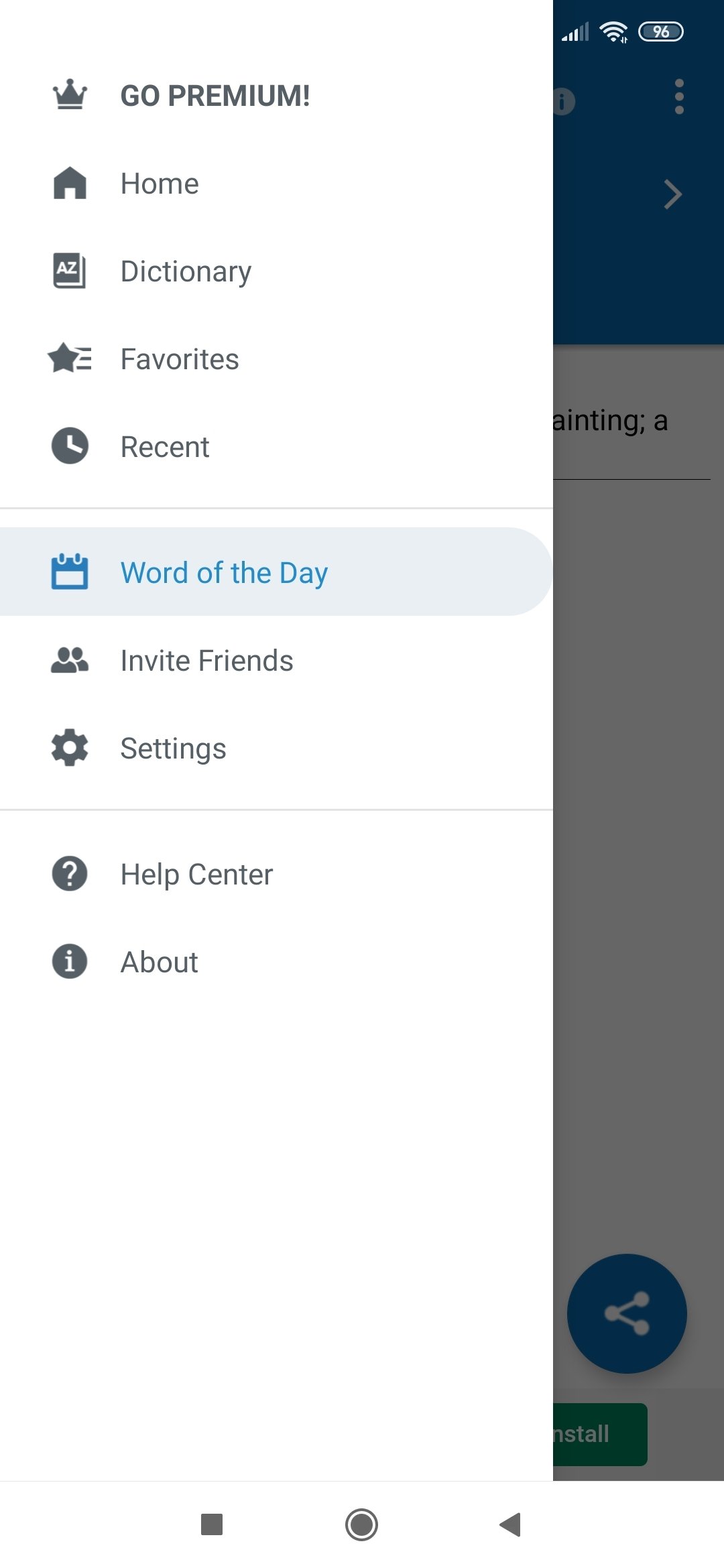This image is a screenshot of the settings or menu page of a dictionary app on an Android smartphone. The menu page, which dominates the screen, features a clean white background with various options displayed. 

At the very top, there's a "Go Premium" option, likely inviting users to subscribe to an ad-free version of the app. Below this, you find a list of navigational options: "Home", "Dictionary", "Favorites", and "Recent". 

The next section includes three more options: "Word of the Day", "Invite Friends", and "Settings". Currently, "Word of the Day" is selected, indicated by its blue text and a grayed-out background highlight.

The final section of the menu presents "Help Center" and "About". At the bottom of the smartphone screen, the conventional Android navigation buttons are visible: the "Tabs" button, the "Home" button, and the "Back" button.

In the background of the menu, there is a hint of the app's interface featuring a blue and white design. Additionally, at the bottom-right corner of the screen, there's a "Share" option and a small green "Install" button, possibly related to additional app content or features.